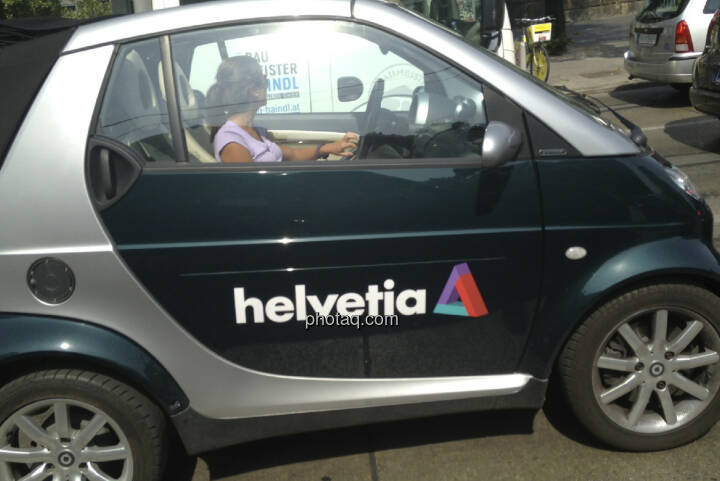A side view of a small electric smart car captures a blonde, caucasian woman with a ponytail driving into a parking lot. Her left hand grips the steering wheel, and she's seen through the closed windows, wearing sunglasses and a lavender T-shirt. The car, tinted in a deep forest green complemented by a silver trim along the sides and bumpers, stands out in the image. Two of its silver-spoked rims are visible. Prominently displayed on the car door is the text "Helvetia," in white Helvetica font, adjacent to a purple, red, and aqua blue three-dimensional triangular logo. Noteworthy is an added URL, "photoac.com," suggesting image copyright.